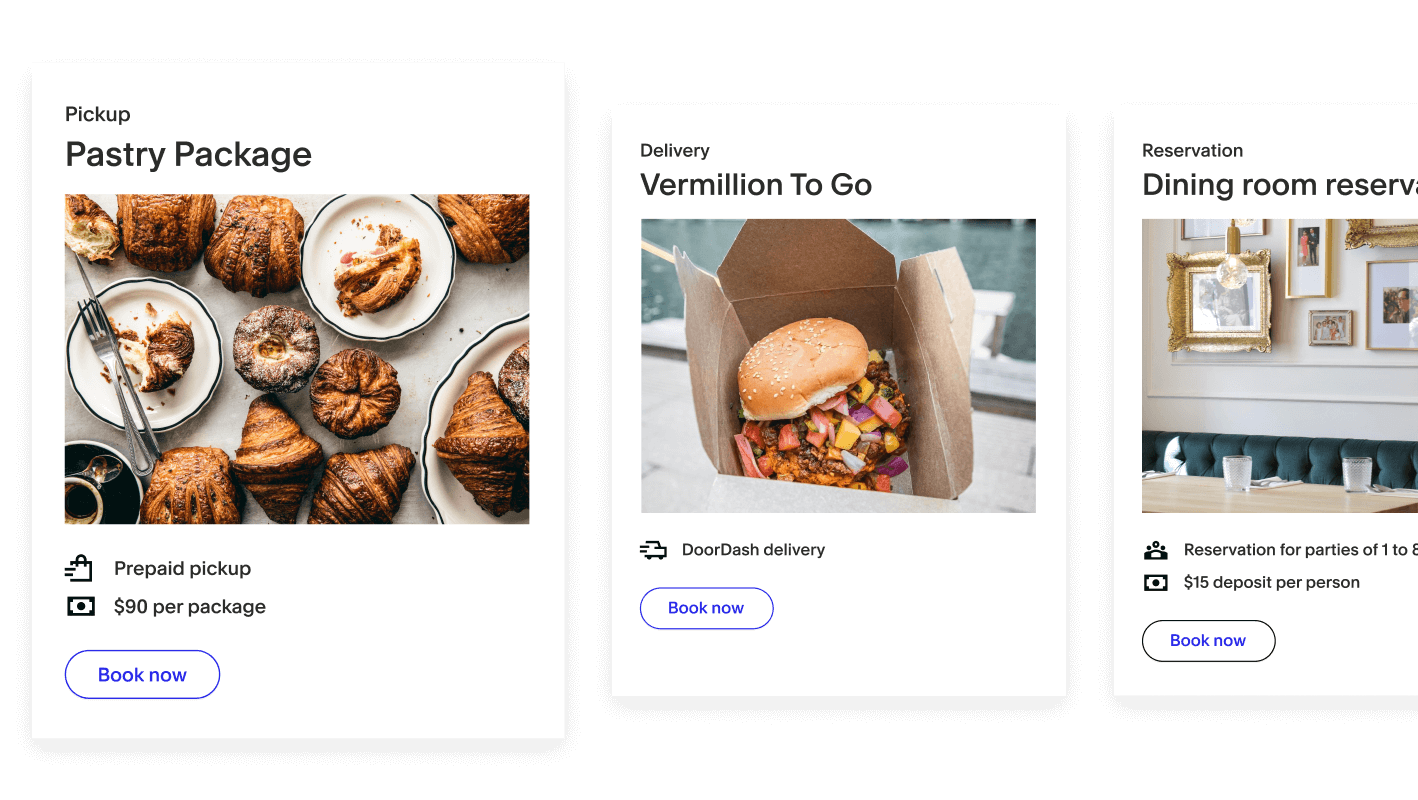A screenshot of three pages showcasing various dining options with food items displayed on each. 

1. The first page features an offering labeled "Pastry Package." It includes an assortment of brown pastries, accompanied by two plates and a fork. The pricing details indicate "$80 per package" with an option to "Book Now" for prepaid pickup.
   
2. The second page is titled "Delivery: Vermilion To-Go," and it depicts a bagel served with fried potatoes and hot dogs. This option is available through DoorDash delivery, with a "Book Now" button prominently displayed.

3. The third page advertises "Reservation: Dining Room." It shows a cozy dining room with a white back wall adorned with pictures, and tables set with cups and plates. The details mention that reservations are available for parties of one to one person, requiring a $15 deposit per person, with the option to "Book Now." 

Each page provides a clear call-to-action to book or reserve their respective services.